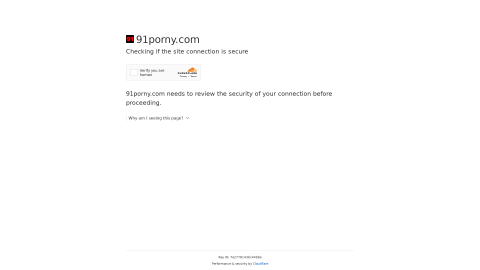The image is a small, hard-to-read screenshot with a predominantly white background. In the top left corner, there's a black box featuring some red elements, though the exact details are unclear due to its size. Adjacent to this box, the text "91POMY.com" appears in black font, and directly beneath it, in a smaller black font, it reads "checking if the site connection is secure."

Below this text, there’s a small gray rectangle housing a white square, which seems like a checkbox option. To the right of this checkbox, there's a distorted icon that is presumably associated with Cloudflare, based on its recognizable shape despite the blurriness.

Further down, in black font, the message "91POMY.com needs to review the security of your connection before proceeding" is displayed. At the very bottom, in a tiny font, there's the clickable text "Why am I receiving this page," inviting users to understand the reason behind this security prompt.